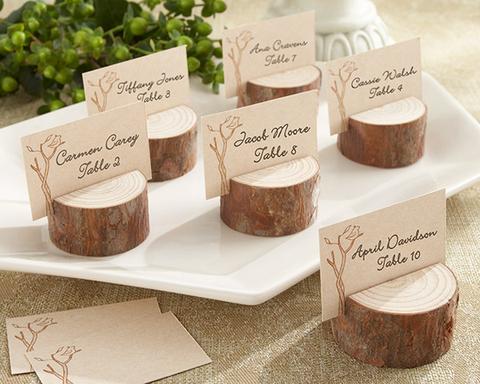In this grainy photograph, a rustic place setting arrangement is meticulously laid out on a brown and white mottled tablecloth. The focal point is a white dish with a trapezoidal shape, occupying the center of the frame. Placed on it are five unique wooden blocks, each fashioned from thin, reddish-brown tree trunk slices with visible growth rings on the cut surface. These wooden blocks, complete with notches, cradle cream-colored paper cards. Each card features a delicate design on the left of a bare tree branch with two leaves and a small bird, alongside a handwritten name and table number on the right. The names and tables include Tiffany Jones at Table 3, Carmen Carey at Table 2, Jake Moore at Table 8, Cassie Walsh at Table 4, and an indistinct name at Table 7. One additional wooden card holder, labeled April Davidson, Table 10, rests on the tablecloth in the bottom right corner. The top left background displays a blurred green clover-like plant, adding a touch of natural charm to the scene.